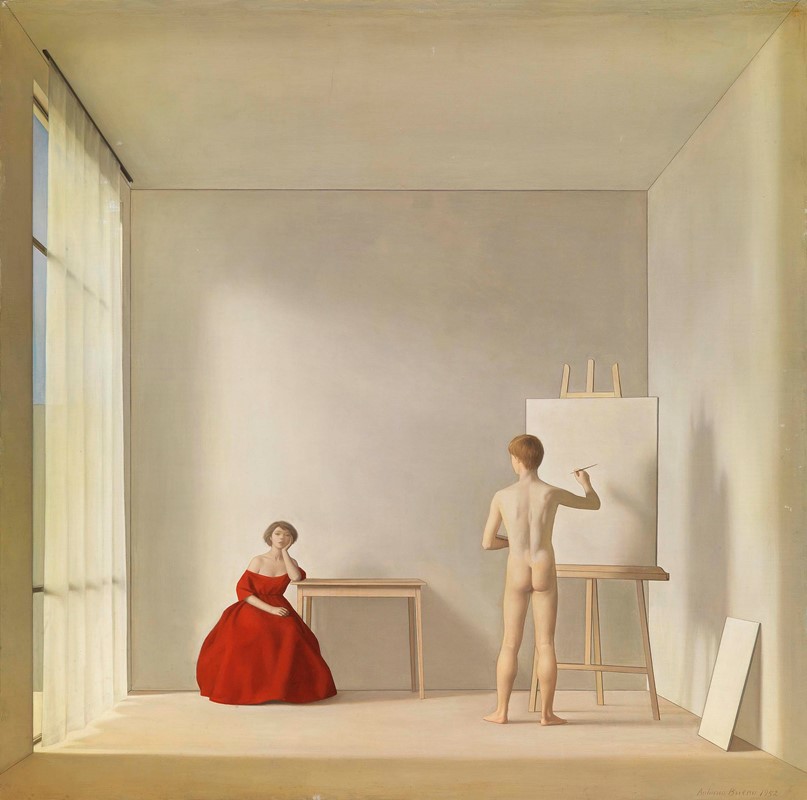This painting depicts a serene and intimate indoor scene centered around two figures. To the left, a woman sits pensively at a wooden table, resting her left arm on the tabletop and cradling her head with her arm. She dons an elegant off-the-shoulder red ball gown, adding a vibrant pop of color to the otherwise muted environment. Sunlight filters gently through a floor-to-ceiling window with white curtains to her left, casting a warm glow into the room. To her right, a nude man stands poised before an easel with a blank canvas, his back to the viewer. His right hand holds a brush aimed at the canvas as his left arm bends at the elbow. The man's shadow is cast on the nearby wall, adding depth to the scene. The room itself is minimalist, painted in subdued tones of white and cream, and the floor appears to be concrete. The only other notable objects are another blank canvas on the floor and the woman's table, emphasizing the artistic and contemplative atmosphere of the space. The overall composition suggests a moment of creative introspection amidst a tranquil setting.